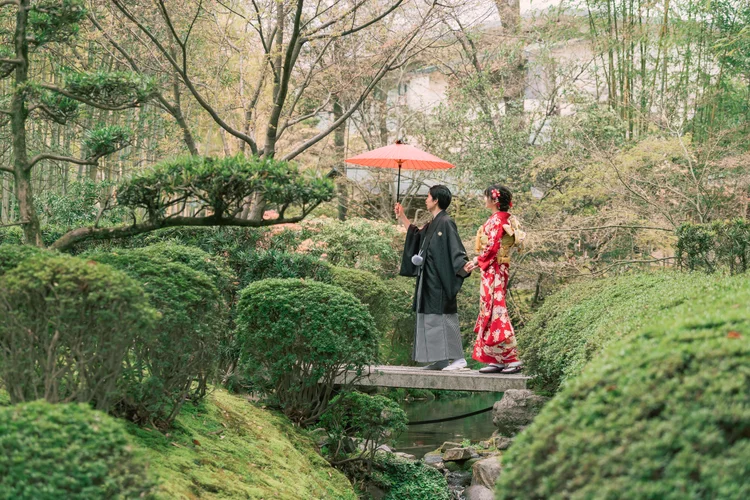This photograph, taken outdoors, captures a serene moment of a Japanese couple as they wander through a dense forest. In the foreground, manicured, rounded bushes and moss-covered rocks add a touch of order amidst the natural setting. The couple is seen crossing a stone bridge over a small creek that runs through the center of the image. The man, dressed in a black kimono and gray pants, holds up a pink umbrella to shield them from the elements. The woman, walking slightly behind him and holding his hand, is adorned in a red dress with a white floral pattern, complemented by traditional Japanese sandals and a red and white flower in her dark hair. Her attire also includes a noticeable accessory on her back, likely part of her traditional costume. All around them, the scenery is lush with green bushes and wild growth of trees. In the far background, partially obscured by the foliage, the vague outline of a house can be discerned. The pale sky peeks through the canopy, creating a calm and timeless atmosphere.